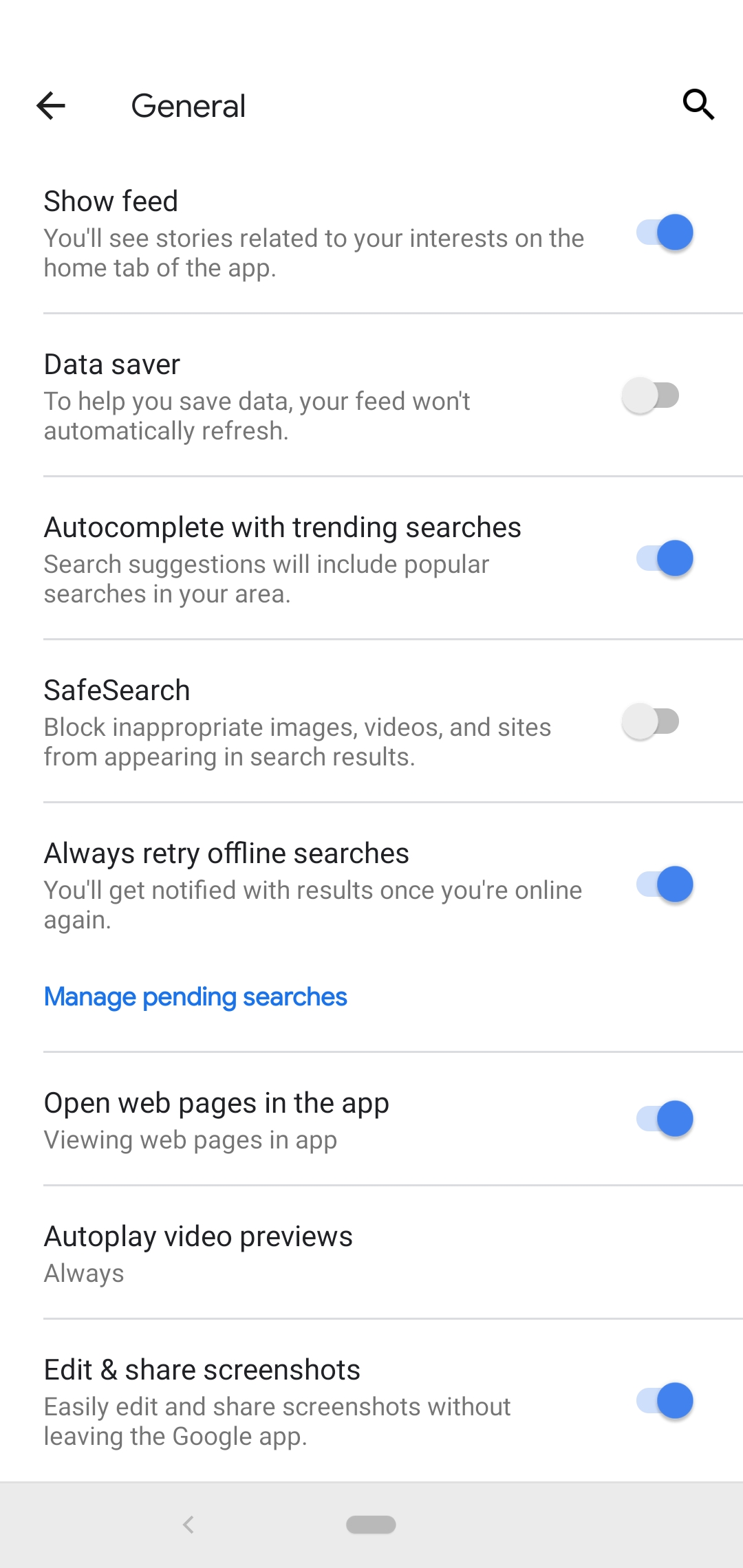A detailed description of the mobile phone UI:

At the top left corner, there is a left-pointing gray arrow, next to which the word "General" is displayed. On the far right, there is a gray magnifying glass icon, indicating a search function. Below, in bold text, it reads "Show Feed," followed by the description, "You'll see stories related to your interests on the home tab of the app." This feature can be toggled on or off, and it is currently switched on.

A faint gray line separates the sections. The next feature is "Data Saver," described as helping to save data by preventing the feed from automatically refreshing. This toggle switch is currently turned off. Another faint gray line follows.

The subsequent feature is "Autocomplete with trending searches," which indicates that search suggestions will include popular searches in your area. This feature is toggled on. A faint gray line divides the sections again.

Next is "Safe Search," described as blocking inappropriate images, videos, and sites from appearing in search results. This toggle switch is currently off. Another faint gray line follows.

The "Always retry offline searches" feature is next, which notifies you with search results once you are online again. This is toggled on, and beneath it is a link in blue text that says "Manage pending searches."

Further down, another faint gray line introduces the "Open webpages in the app" feature, described as allowing the viewing of webpages within the app. This switch is toggled on. 

Following this is "Auto-play video previews," set to "Always." There is no toggle switch for this feature, and it is followed by another faint gray line.

The next feature is "Edit and share screenshots," which facilitates easy editing and sharing of screenshots without leaving the Google app. This switch is turned on as well.

At the bottom, there is a gray bar with an oval-shaped darker gray button in its center. To the left of this button, there is another left-pointing arrow.

This detailed description captures all elements and functionalities present in the UI.